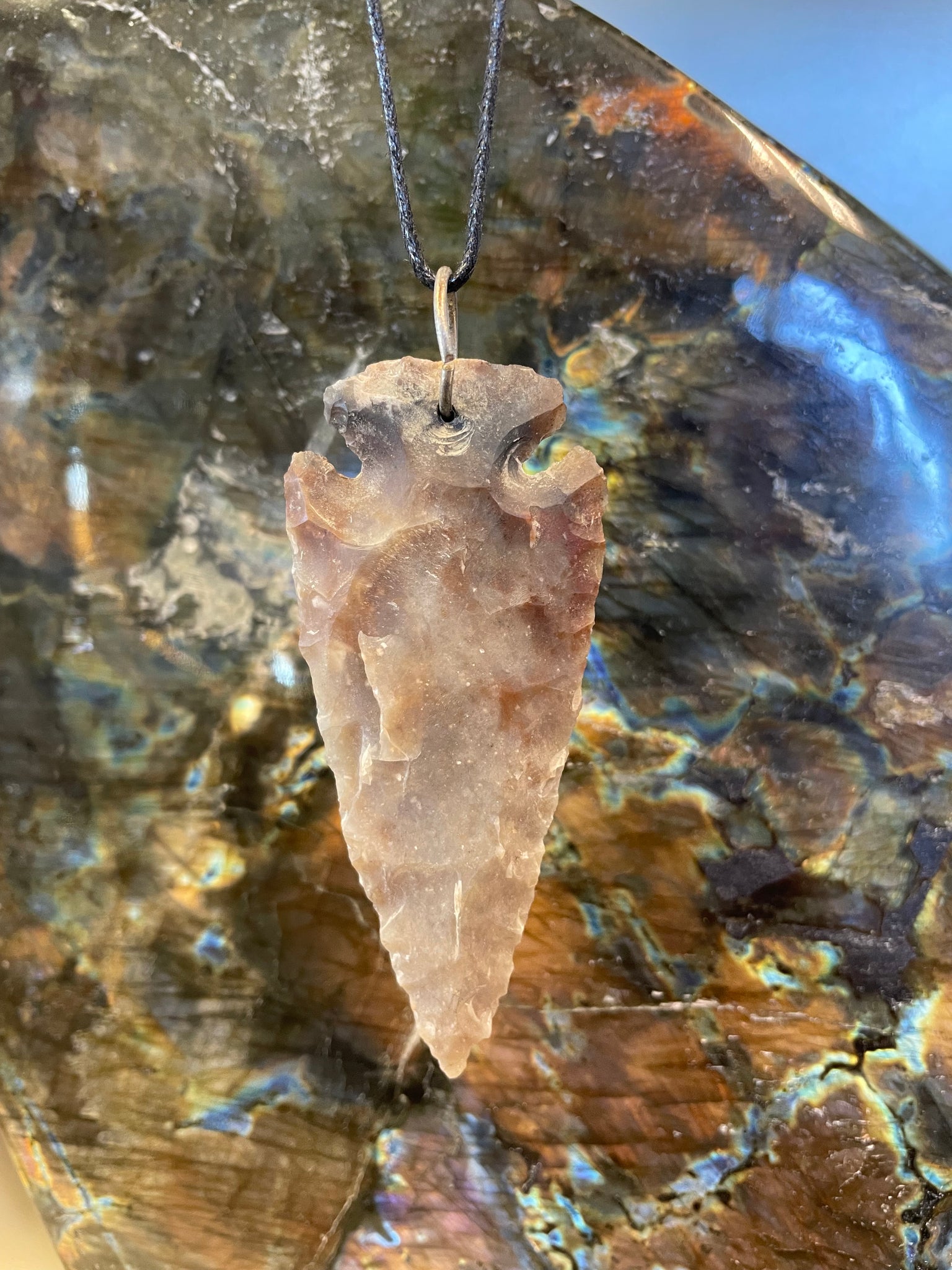This detailed color photograph showcases a traditional-style arrowhead, seemingly a recent recreation, likely intended for product photography, possibly for an Etsy listing. The arrowhead is crafted from a pinkish stone and exhibits hand-chipped, slightly ragged edges that suggest a rough texture. It comes to a sharp point at the bottom and has scattered white specks on its surface. A silver metal ring secures the arrowhead, attaching it to a black leather cord. The arrowhead is displayed against a polished stone backdrop featuring splotches of yellow, brown, and blue, with various mineral streaks and features. In the upper right-hand corner, a blue background is partially visible, enhancing the contrast between the dull, rough arrowhead and the shiny, polished stone beneath it. The entire composition emphasizes the natural, rustic aesthetic of the stone arrowhead pendant.